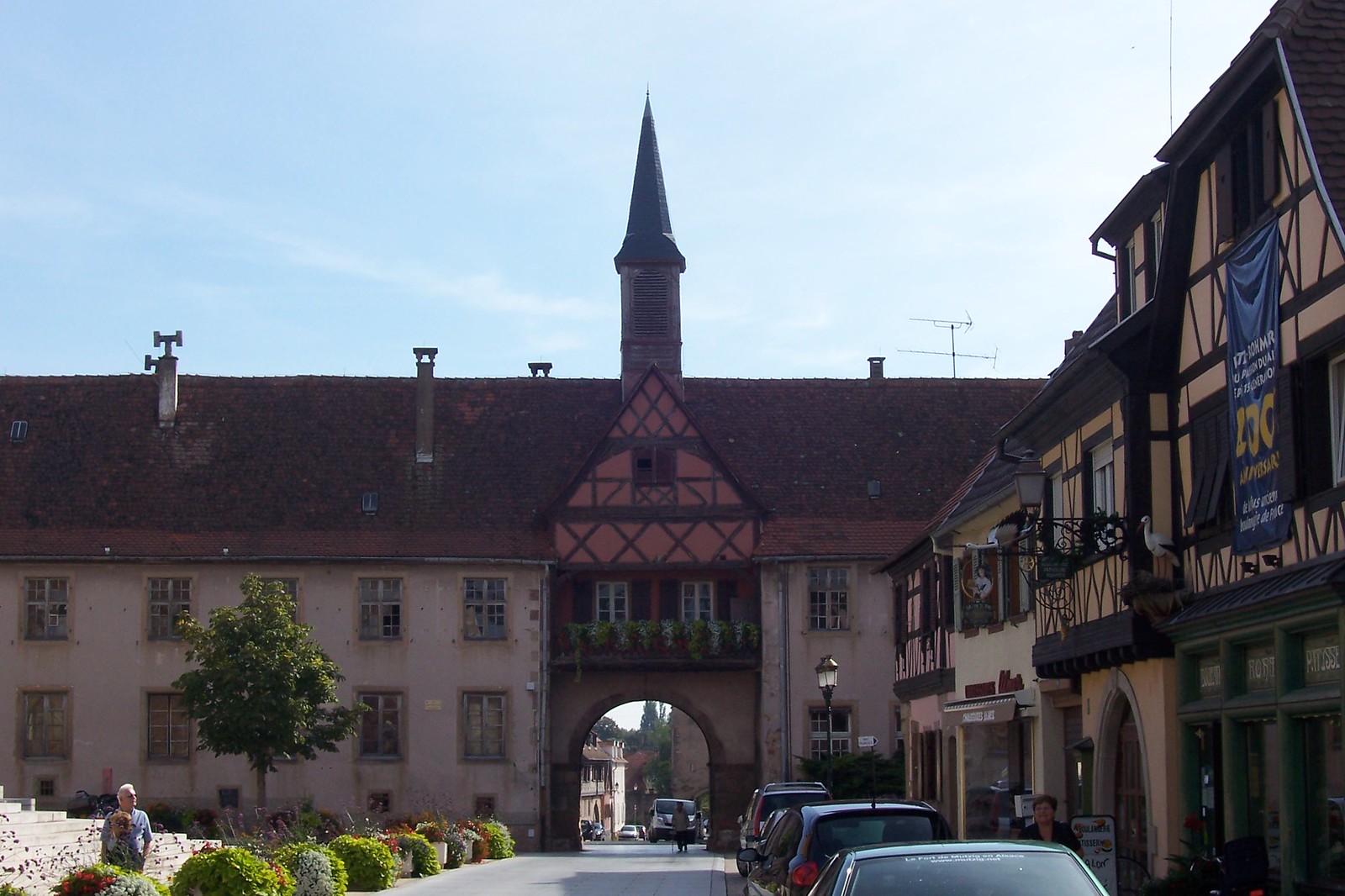The photograph captures an old European-style building prominently situated along the bottom and right-hand side of the frame, characterized by its browns and tans. The structure features numerous windows and archways, with a central archway through which a road passes. The bottom center of the image showcases this road as it extends through the archway and into a network of other buildings and roads visible beyond. To the right of the building, several cars are parked, while on the left-hand side, bushes and shrubs are interspersed with trees. A person stands in the left-hand corner of the scene, gazing up at the building. A sign or banner is draped on the left side of one of the buildings. In the background, a tall tower rises prominently, and there are faint indications of smokestacks among the trees. The sky above is a vibrant blue with scattered cloud coverage, contributing to the picturesque quality of what appears to be a quaint European city setting.